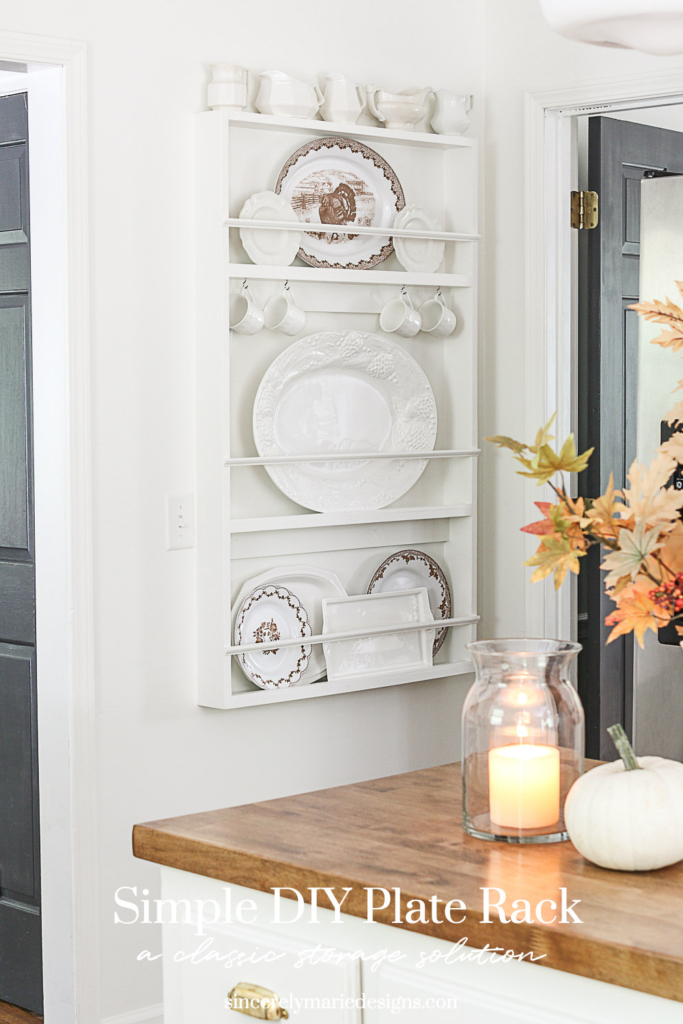This photograph captures a meticulously arranged kitchen scene centered around a mounted plate rack, labeled at the bottom as "Simple DIY Plate Rack, a Classic Storage Solution." The plate rack is mounted on a white wall and displays an array of kitchenware. The top shelf is home to a collection of white teapots, sugar bowls, and a decorative plate with a brown edge and design. The second shelf features vertically displayed plates and small white pitchers, while the third shelf showcases a large serving plate and four hanging cups. The bottom shelf holds more plates with brown designs and a central serving tray. Rails across each shelf secure the items in place.

In the foreground to the lower right, a white kitchen island with a butcher block wooden countertop is visible. Adorning this countertop are seasonal decorations, including a white painted gourd, a vase containing autumn leaves, and a glass jar holding a lit candle. The kitchen area also features white cupboards with gold pulls beneath the counter. Two black doors can be seen - one likely leading to a pantry.

Overall, this image highlights a harmonious blend of functionality and aesthetic charm, showcasing the plate rack as both a practical storage solution and a focal decorative element.